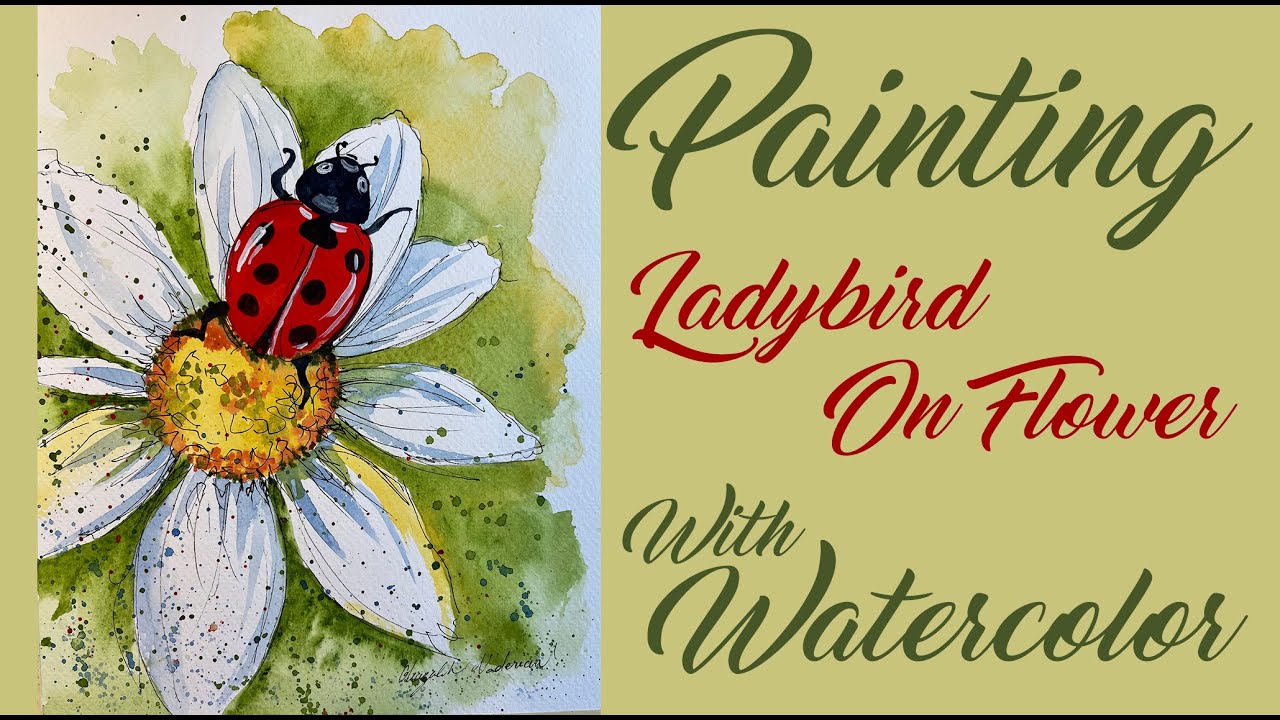This captivating image, resembling a postcard or an ad, features a beautifully detailed watercolor painting of a ladybug on a daisy. The left side of the image showcases the vibrant artwork: a large ladybug with a red shell adorned with black spots crawls atop the daisy, which is intriguingly white with a yellow center. Surrounding the flower, hints of green suggest the natural foliage, while darker green splotches are artistically scattered across the scene for added effect.

On the right side, elegantly cursive lettering provides context to the artwork. In green, it reads "painting," followed in red by "ladybird on flower," and beneath that, again in green, "with watercolor." The background behind these words is a soothing yellowish cream, which complements the painting and enhances its postcard-like charm. The entire piece, vertically oriented, exudes a harmonious blend of artistic creativity and nature's beauty.